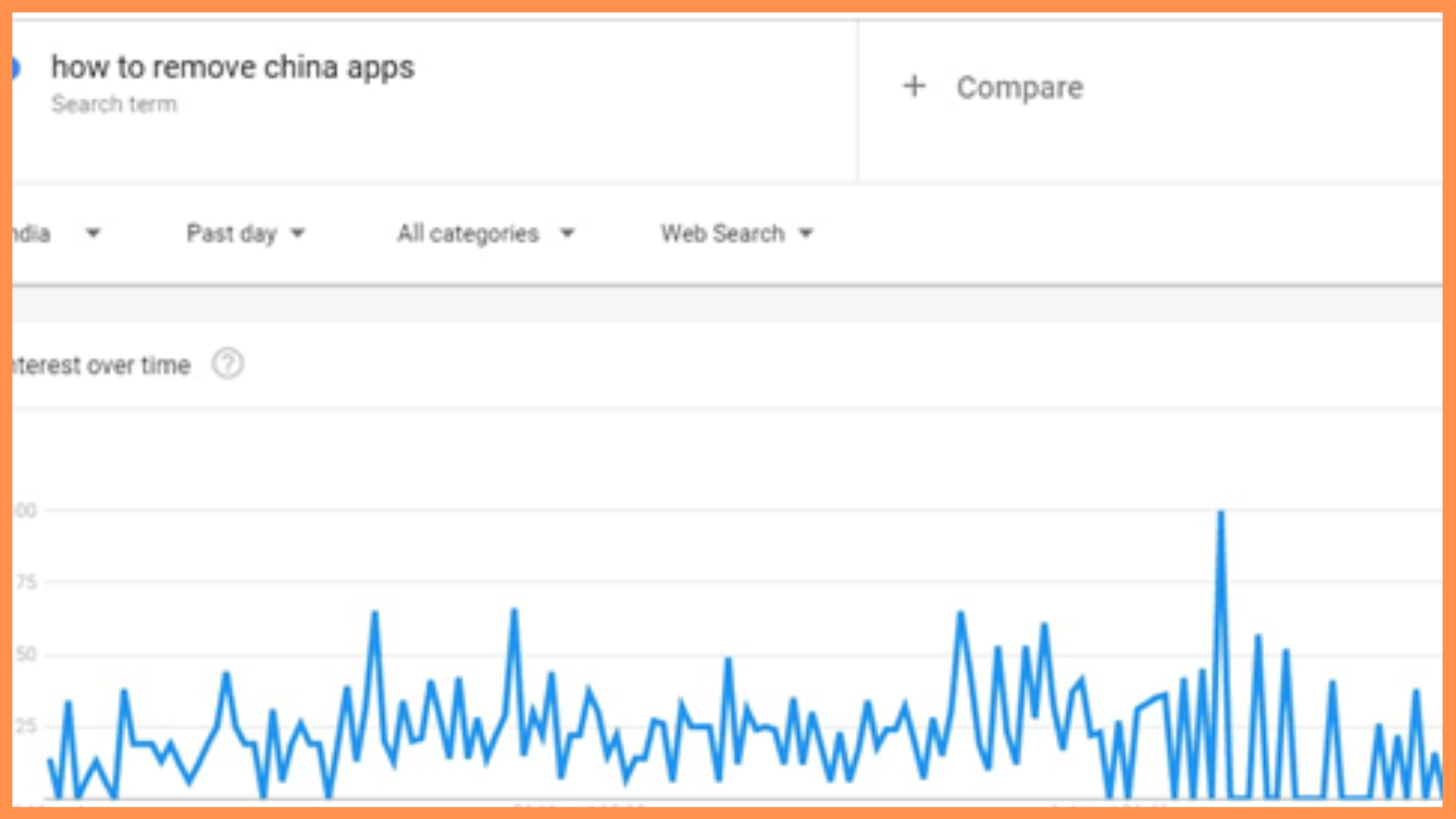This image is a partial screenshot of a data visualization chart, encapsulated within a thick orange border. The main section of the chart is segmented into various boxes and labels. At the top-left corner, there is a text box titled "How to Remove China Apps" in bold black font, followed by a description in gray text that reads "search term" inside a rectangular box. Adjacent to this box, on the left side, is a smaller box with a plus sign labeled "compare."

Beneath these texts is a navigation bar containing multiple drop-down menus. The first drop-down menu shows a truncated search term, with visible letters "N DIA" and a small downward-pointing arrow. Next to it, another drop-down menu displays "Past day" with a similar arrow. This is followed by "All categories" and "Web search," both accompanied by drop-down arrows.

Directly below the navigation bar is a light gray separator line, under which lies the main chart area. The chart appears as a line graph with fluctuating data points, resembling the patterns of a heartbeat monitor. It includes a title "Interest Over Time," accompanied by an informational circle with a question mark.

The chart has five horizontal gray lines, with the top line stretching across the width of the chart and the subsequent four marked with numerical values: 100 at the top, followed by 75, 50, and 25 descending respectively. A blue line traverses the chart, spiking and dipping to represent variations in recorded interest. The peaks and troughs of this blue line range from highs of 100 to lows just below 25.

The overall background of the image is white, highlighting the colorful elements and text prominently.